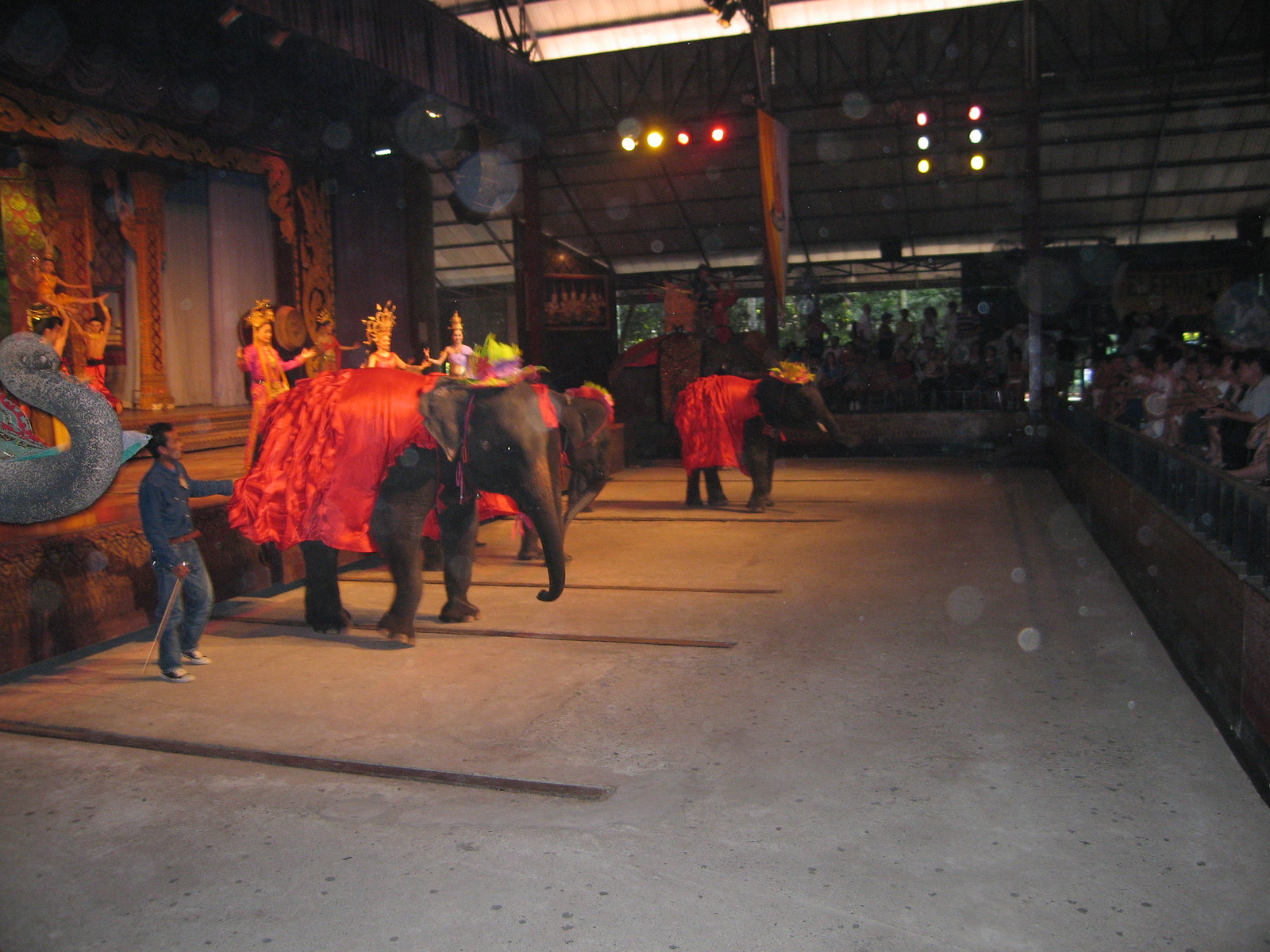This detailed photograph captures an outdoor cultural event featuring a vibrant performance with Indian elephants and elaborately dressed participants. At the forefront, there are four elephants adorned with red silk drapes over their backs and bright, colorful hats in shades of red and yellow. A man dressed in blue jeans and a matching shirt stands next to the elephants, holding a stick. The background reveals a stage to the left with three women dressed in brightly colored outfits of pink, purple, and red, each wearing ornate golden headdresses. In addition, there are statues and props adding to the decorative setting. Behind a fence, a crowd watches the performance, some seated in stands under a roof with spotlights illuminating the scene. The setting is populated with greenery, contributing to the outdoor ambiance. The combination of the elephants, the performers in their ornate attire, and the cheering crowd suggests this is a cultural festival or ceremonial event, richly detailed in its presentation.